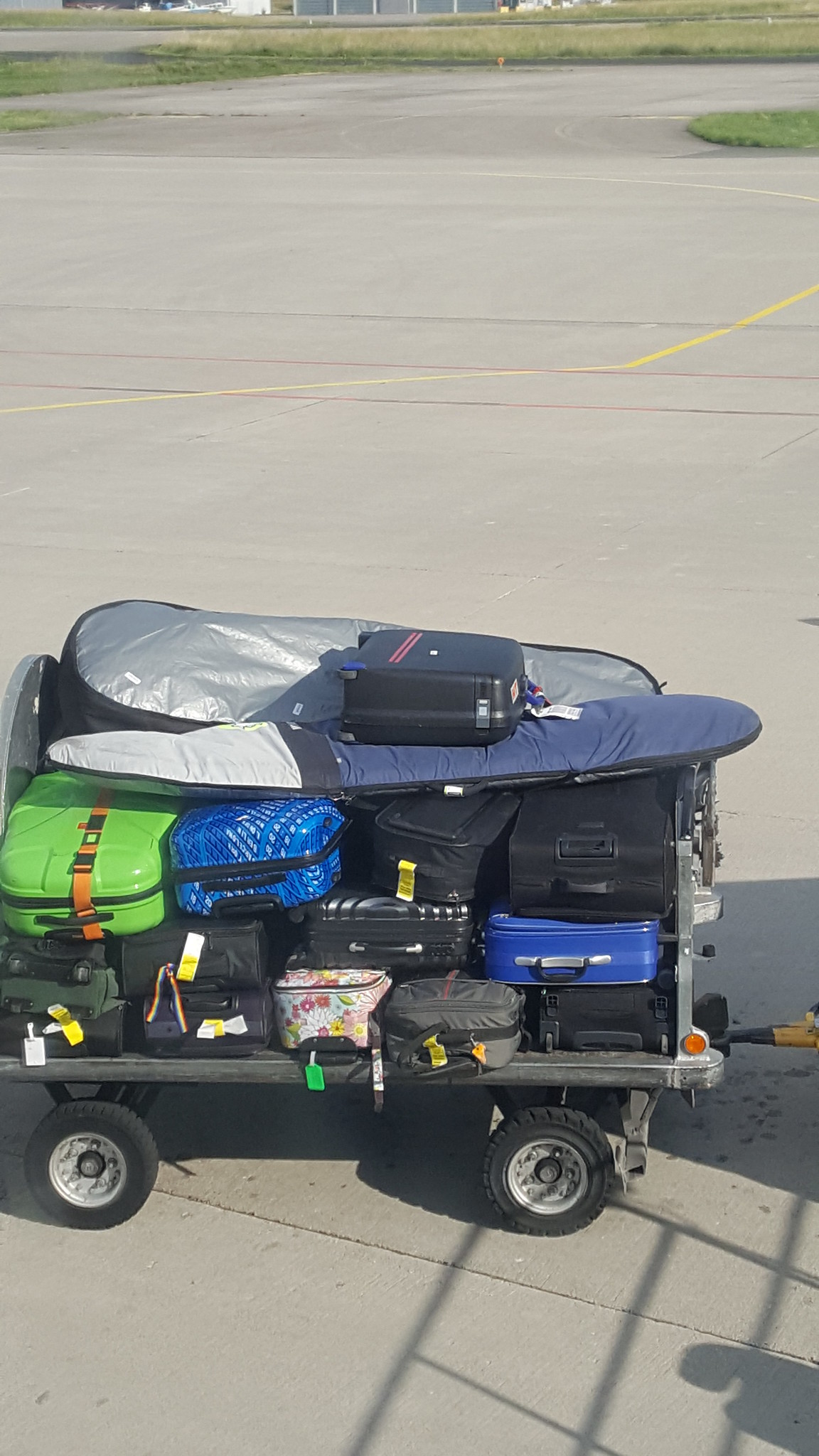This photograph, taken on a sunny day at an airport, features a luggage trolley on the tarmac, loaded with various pieces of luggage. The steel cart, characterized by its open sides, rugged rubber-tired wheels, and distinct yellow and red paint lines on the ground, is centrally positioned in the frame. The trolley is stacked with a mix of 14 hard-shelled and soft-sided suitcases, mostly black, but with notable exceptions including a hard-shelled lime green suitcase, two blue suitcases—one hard and one cloth—and a distinctive white bag adorned with flowers. At the very top of the stack are two elongated objects, likely surfboards or a guitar case, with a smaller black suitcase perched on top of them. In the rear background, part of a plane wing is barely visible, suggesting proximity to the aircraft. The scene is also bordered by a parking area and patches of grass, adding to the airport setting. Bright sunlight casts clear shadows, underscoring the high sun and clear weather conditions.